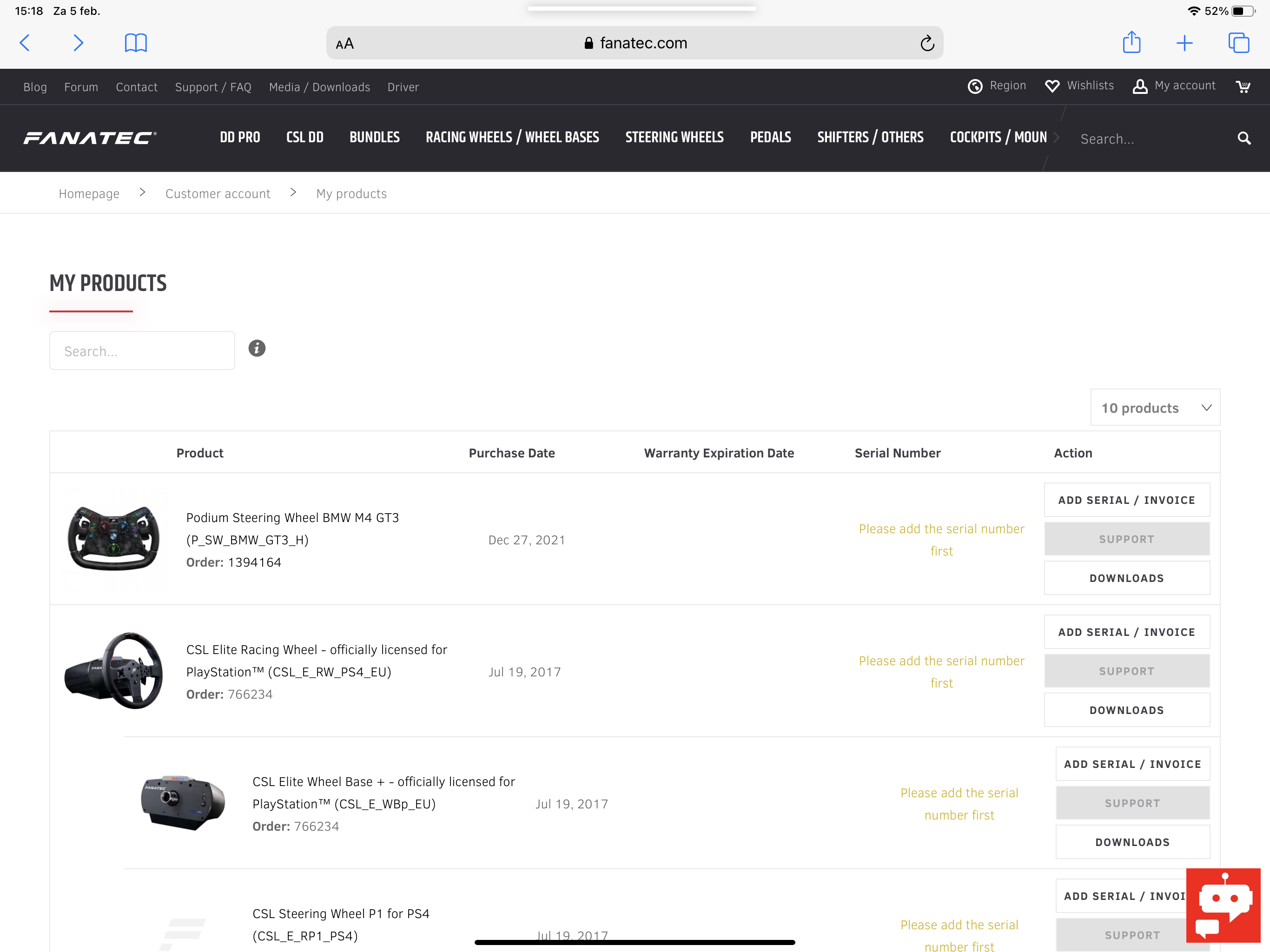This image is a screenshot captured from an Apple device, likely a tablet, as evidenced by the displayed Wi-Fi signal, battery icon, time, and calendar date at the top of the screen. The screenshot showcases a webpage opened to fanatec.com, a site dedicated to racing simulation hardware.

The site features a clean, user-friendly design with a white background and a prominent black navigation bar. Navigation options include "Blog," "Forum," "Contact Support," "FAQ," "Media Downloads," and "Drivers." Additionally, users can select their region, view their wishlist, create a new account, and access their shopping cart.

Detailed catalog tabs on the website include "DD Pro," "CSO DG," "Bundles," "Racing Wheels and Wheel Bases," "Steering Wheels," "Pedals," "Shifters," "Others," "Cockpits," and "Mounts."

The customer account shown in the screenshot lists products ordered in the years 2017 and 2021. The ordered items include a steering wheel, a racing wheel, an elite wheelbase, and another steering wheel, all presumably compatible with PlayStation consoles such as PS1 and PS4, indicating a focus on gaming.